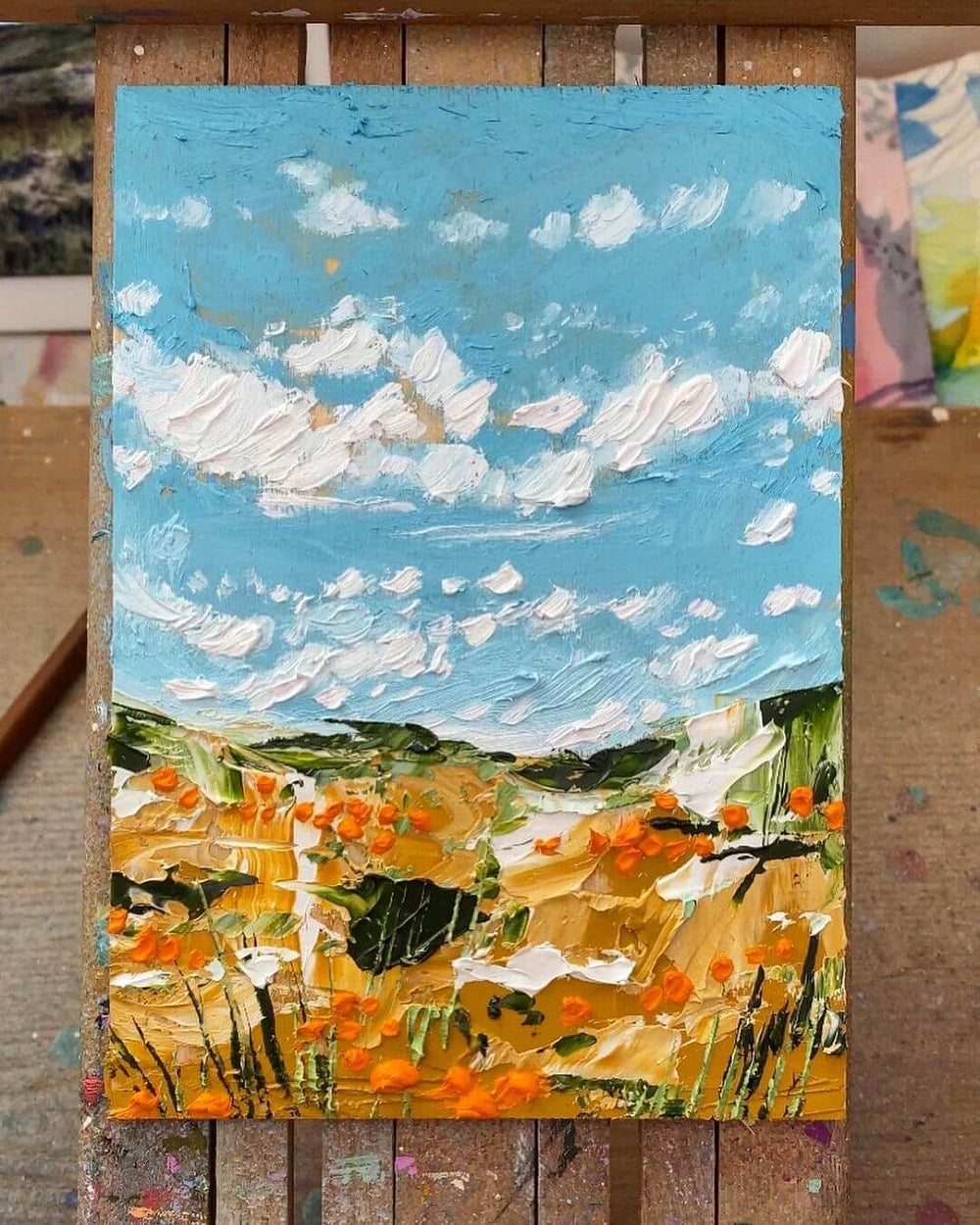This detailed oil painting, likely done on stretched canvas, showcases a captivating outdoor scenery, blending elements of abstract and realistic art. The painting illustrates a vast field, which may resemble a desert or wild countryside, dominated by a striking blue sky filled with thick, white, impasto clouds. The clouds are created using noticeable globs of paint, adding texture and depth to the sky.

Two-thirds down the painting, the horizon meets the ground, transitioning into rolling green hills. The foreground bursts with vibrant wildflowers, their green stems standing out amidst shades of orange, tan, and yellow. The flowers, possibly resembling tiny poppies, are depicted in vivid reds and oranges, adding a delightful contrast to the golden grass below. Additionally, the lower part of the painting features yellow spots and green, reed-like markings, enhancing the sense of a dense, lush landscape. 

This artwork, hanging on a wall surrounded by other vivid paintings, remains enigmatic—its modern, hand-painted style could be either a child's imaginative creation or an artist's abstract portrayal of natural beauty.